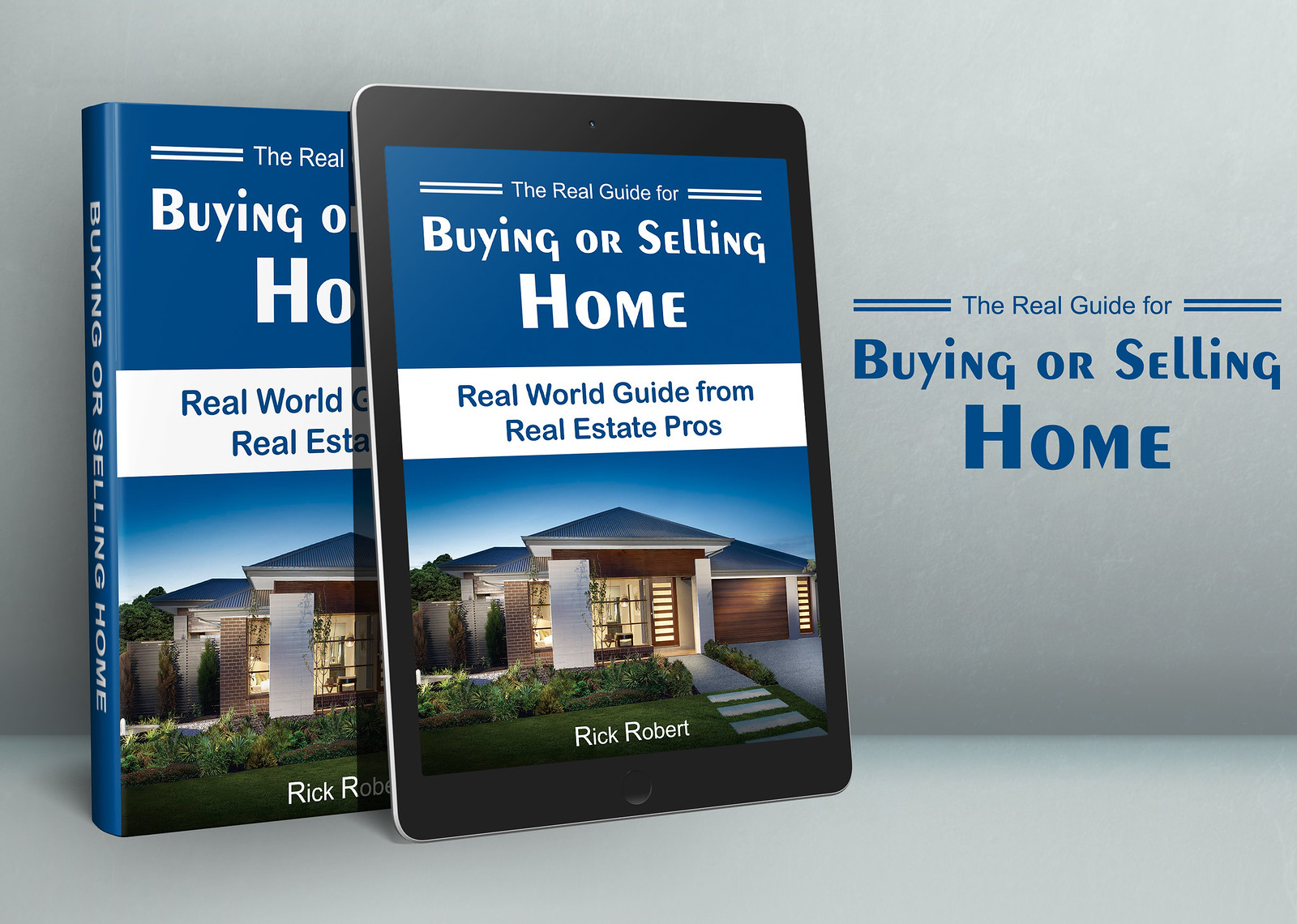The image is an advertisement for a real estate guide titled "The Real Guide for Buying or Selling Home, Real World Guide from Real Estate Pros" by Rick Robert. Central to the image is a black tablet, displaying the guide's cover featuring a well-lit house at dusk. To the left of the tablet is the physical book copy of the guide. The tablet and book slightly lean against each other, both facing towards the right. A gradient gray background enhances the blue text on the right side of the image, reiterating the guide's title. The visual composition is accentuated with a subtle shine emanating from the upper left side of the screen, illuminating the scene. The color scheme includes various shades of blue, black, gray, and lighter brown elements, underscoring the professional and polished look of the advertisement.